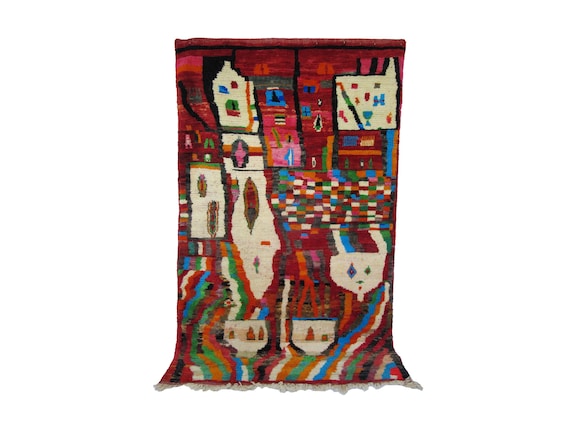The image portrays a highly detailed and vibrant knitted or woven textile, possibly a rug, tapestry, or blanket, displayed on the floor, adding a unique touch to the space. The textile is saturated with bright and varied colors including reds, blues, greens, yellows, browns, oranges, and dark reds, creating a striking visual impact. It features an abstract and somewhat surreal cityscape, characterized by a patchwork of different building shapes and sizes. 

On the right side of the textile, a cluster of multicolored squares—predominantly featuring whites, blues, greens, yellows, and reds—creates a sense of urban density. Adjacent to these squares, especially to the left, are elongated buildings and other structures that appear to be intricately upside down or mirrored, contributing to a disorienting yet captivating perspective. The bottom section of the textile continues this architectural theme but shows smaller, upside-down houses against a backdrop rich in blue hues.

Amidst this architectural motif, the textile is segmented into three distinct sections, with a central band featuring rectangles filled with a blend of blues, reds, oranges, browns, and whites, adding depth and complexity to the design. Scattered throughout are shapes such as squares, ovals, chalices, and triangles, each hosting their own color combinations of blues and reds. The entire scene is framed against a checkered floor pattern composed of white, red, black, and green hues, enhancing the overall sense of a colorful and eclectic environment.